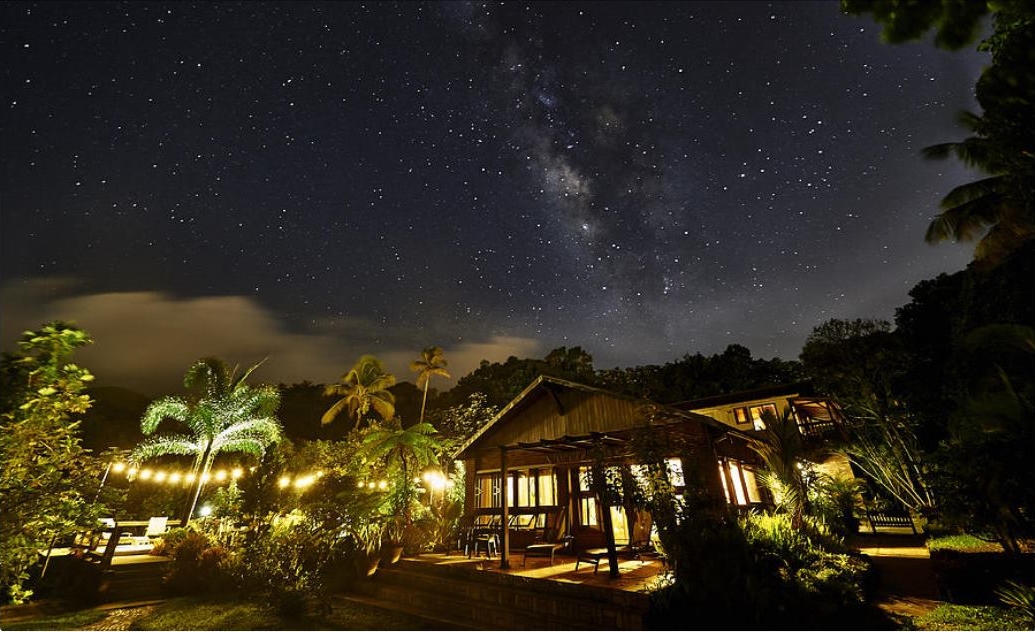This color photograph, likely taken with a wide-angle lens, captures an enchanting night scene of a rustic vacation cabin enveloped in abundant greenery, including lush palm trees and various plants. The cabin, possibly serving as a cozy retreat, is brightly lit from within, casting a warm, yellow glow that spills out through numerous windows and lights up the surrounding area. The structure appears to have a distinct front and back section, creating a layered, inviting layout. 

A spacious patio features several white chairs, which are positioned near a pool situated to the left of the frame, further adding to the leisurely atmosphere. The pool area is outlined by lights arranged in a square formation, enhancing the image's illumination and visual appeal. The sky above the scene, transitioning into night, is adorned with a scattering of stars and subtle, light clouds that only amplify the magical ambiance. The twinkling stars and the cabin’s lights create a striking contrast against the backdrop of the darkened sky, giving the photograph a lively yet serene feel, perfect for a magazine spread showcasing idyllic vacation destinations.